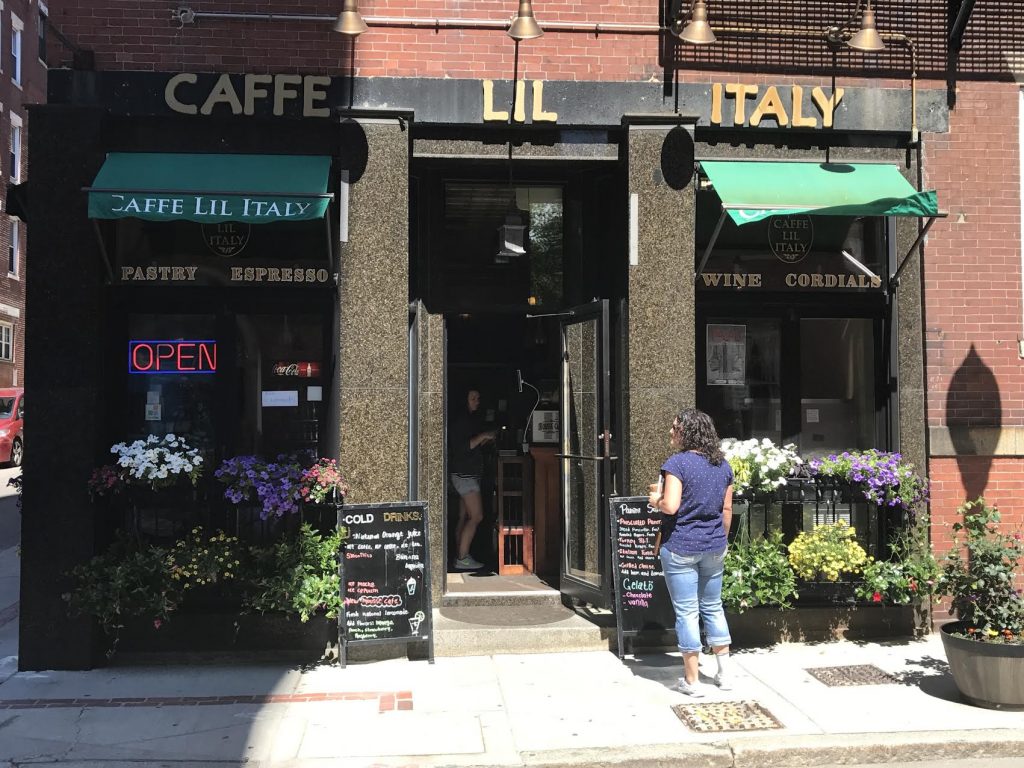This vibrant photograph captures the bustling front entrance of Cafe Lil Italy, a charming local cafe that exudes a welcoming atmosphere. The facade showcases elegant gold lettering on a black beam displaying the cafe's name, "Cafe Lil Italy." Flanking the entrance are two green awnings, also emblazoned with the cafe's name and advertising their delightful offerings: pastry, espresso, wine, and cordials. The entryway is accentuated by rectangular gray stone columns rising up to about 20 feet, lending a grandiose touch to the exterior.

The cafe's front is adorned with an array of colorful plants and flowers nestled in planters that extend up to four to five feet, bringing a burst of nature to the urban setting. Large glass windows, trimmed in dark colors, offer a glimpse into the cozy interior where customers are seen enjoying their drinks and pastries. Outside, a woman dressed in high-rise jeans and a blue shirt stands holding a coffee in her left hand, gazing thoughtfully at the chalkboard menus. These menus, written in vibrant chalk, highlight the cafe's enticing offerings, including 'cold drinks' and other popular items. A neon "open" sign adds a touch of welcoming light to the scene, inviting passersby to step inside and experience the bustling yet homely atmosphere of Cafe Lil Italy.